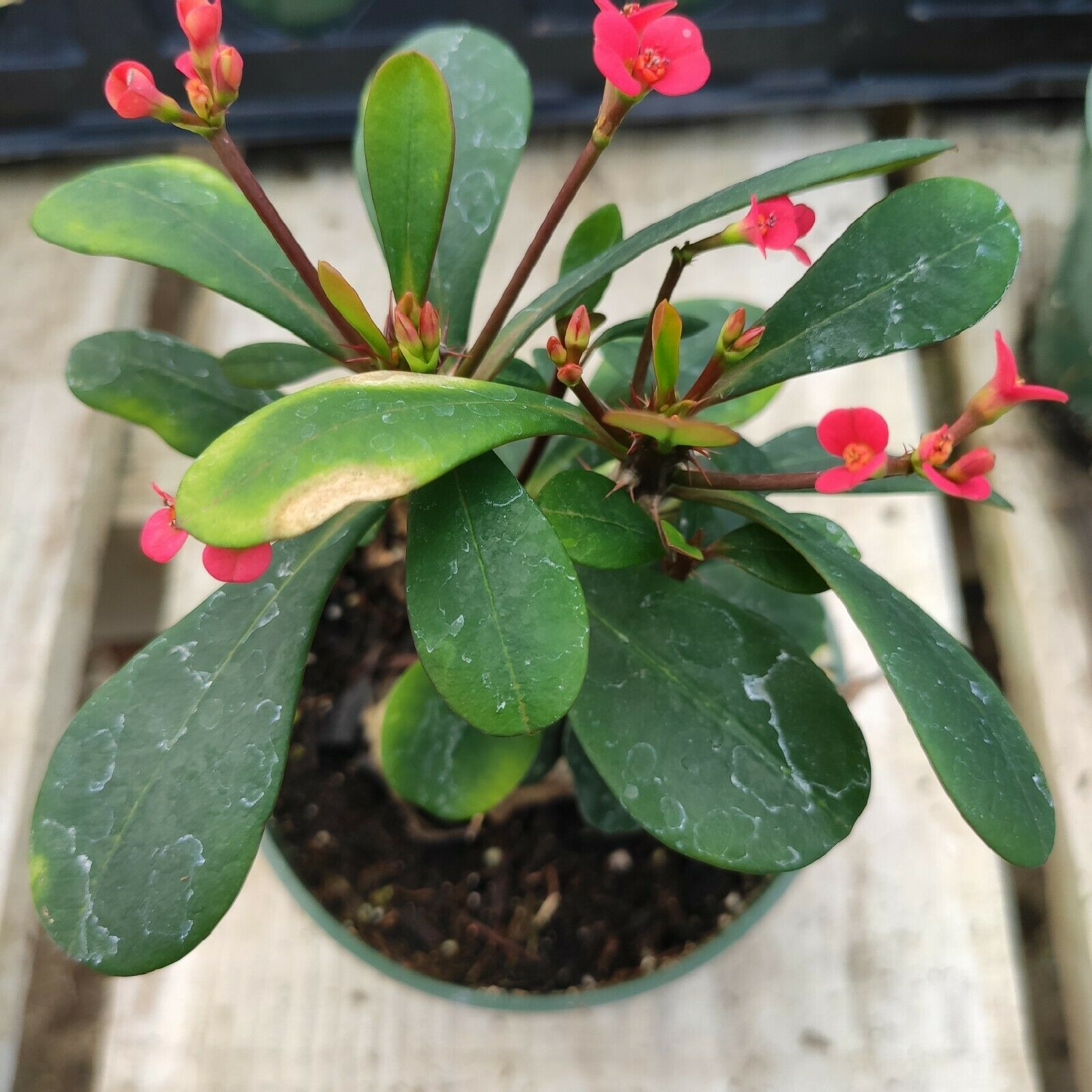This is a detailed photograph taken from above of a potted plant situated on what appears to be a white wooden board. The plant resides in a green pot filled with dark soil. The plant features numerous large, thick green leaves that are broad and oblong, resembling tongues, and some of these leaves display signs of wear, with brown edges as if affected by harsh weather. Notably, the leaves have distinctive white veins. From the base, long stalks rise, bearing small red flowers, each consisting of two prominent petals. Some of these buds have developed into small pink flowers visible behind the green leaves. The background includes a hint of black plastic, possibly related to gardening, further adding depth to the image. Overall, the plant appears generally healthy despite minor imperfections.